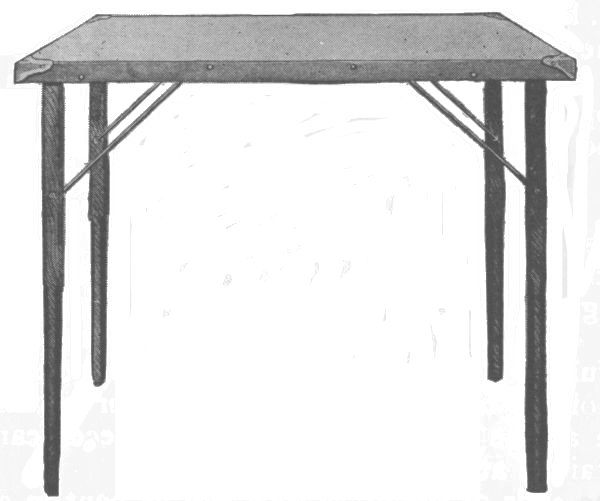This detailed grayscale image appears to be a meticulously drawn representation, likely executed with either colored pencils or graphite. The main subject of the image is a square folding table that is fully unfolded, standing on its four legs. The table's legs and support mechanisms are clearly visible, showcasing the brace attachments to the tabletop. The tabletop itself is light gray with protective metal corner pieces, designed to prevent injury or wear. The legs, which are black, appear to be constructed from plastic. The background of the image is a plain white with subtle gray streaks, providing a minimalistic setting that further emphasizes the table. The entire composition gives the impression of a detailed line drawing or an aged black-and-white photo, rather than a modern photograph, with some specks and imperfections adding to the overall realism and texture of the depicted table.